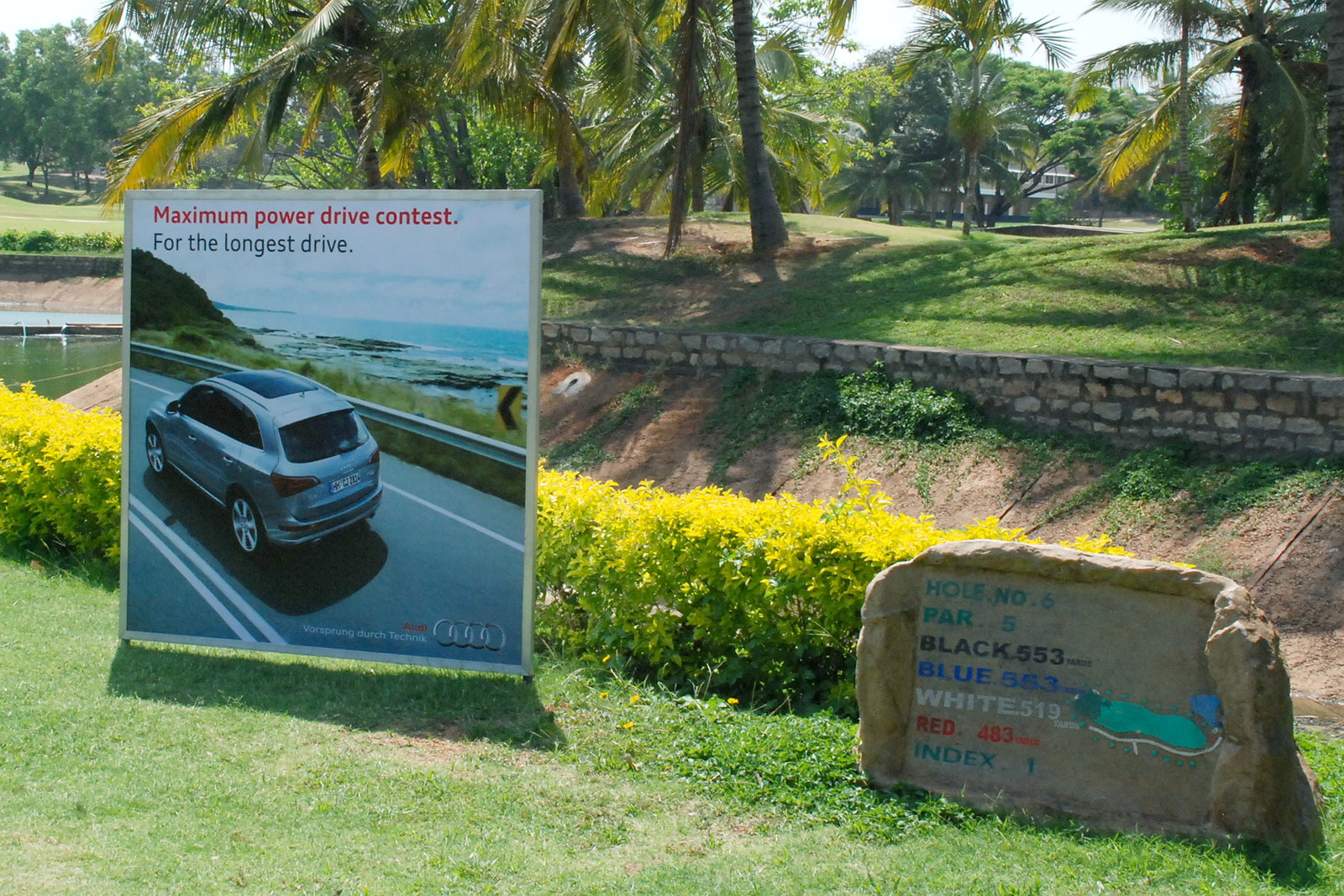This outdoor photograph depicts a scenic tropical section of a golf course. Dominated by numerous palm trees and sandy areas around the trees, the setting includes a well-maintained lawn and a small creek that runs through the green landscape. Prominently displayed in the foreground is a dual set of signs: on the left, a yard-style advertisement for Audi, showcasing an SUV driving along a coastal highway with the ocean in the background. The text on the ad reads "Maximum Power Drive Contest" in bold red, followed by "for the longest drive" below it. To the right of this ad, a stone sign provides detailed information about the golf hole, stating "Hole Number 6, Par 5" with various tee distances listed—black 553, blue 553, white 519, red 483, and an index of 1. Nearby, a small, meticulously designed stone wall flanks the area, adding to the picturesque and organized appeal of the golf course terrain.